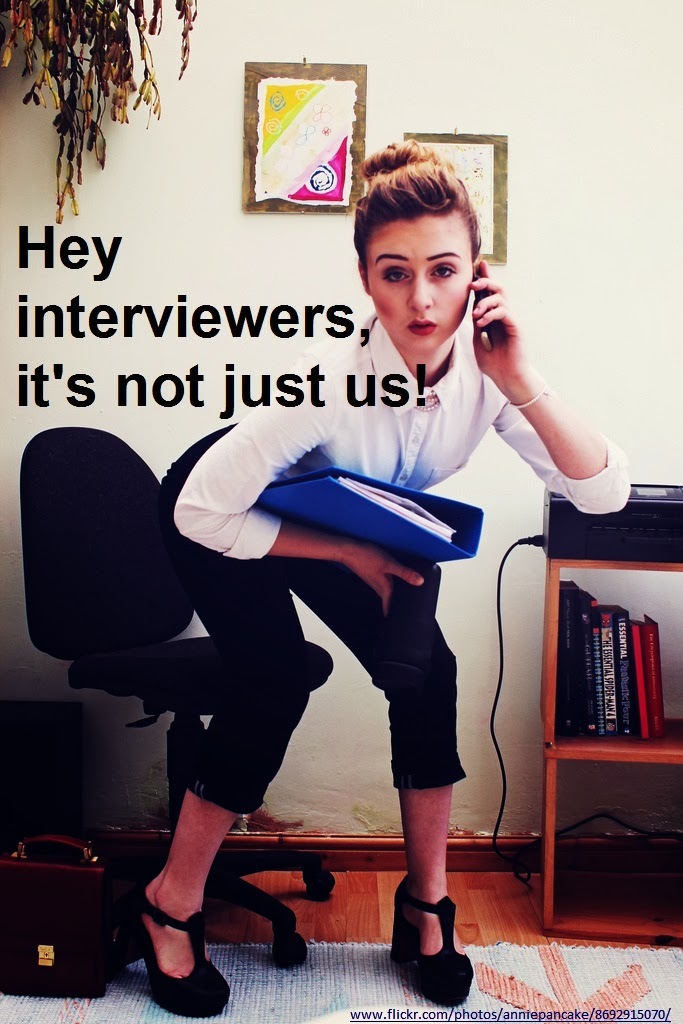The photograph, captured in an indoor office setting, depicts a young blonde woman in her 20s with her hair pulled up in a bun. She wears a white long-sleeve button-up dress shirt, black capris that reach her calves, and high-heeled black platform shoes. The woman is crouched over, as if about to sit or stand up from a black, armless office chair behind her. She holds a blue three-ring binder close to her body in her right hand while holding a cell phone to her ear with her left hand. Her expression appears worried, and she looks directly at the camera.

The setting includes a hardwood floor covered by a pink and white rug. To the right, there is a bookcase with books and a printer on top, and above the woman, a hanging plant is visible in the top left-hand corner. Behind her on the white wall are two colorful posters—one in orange, green, white, and purple. A black purse lies on the floor in the top left-hand corner. The image also contains the text "Hey interviewers, it's not just us," emphasizing the theme of the ad or meme. At the bottom, a website URL reads "www.flickr.com/photos/adforpancake/869-29-15070," indicating a screen dump from a website.